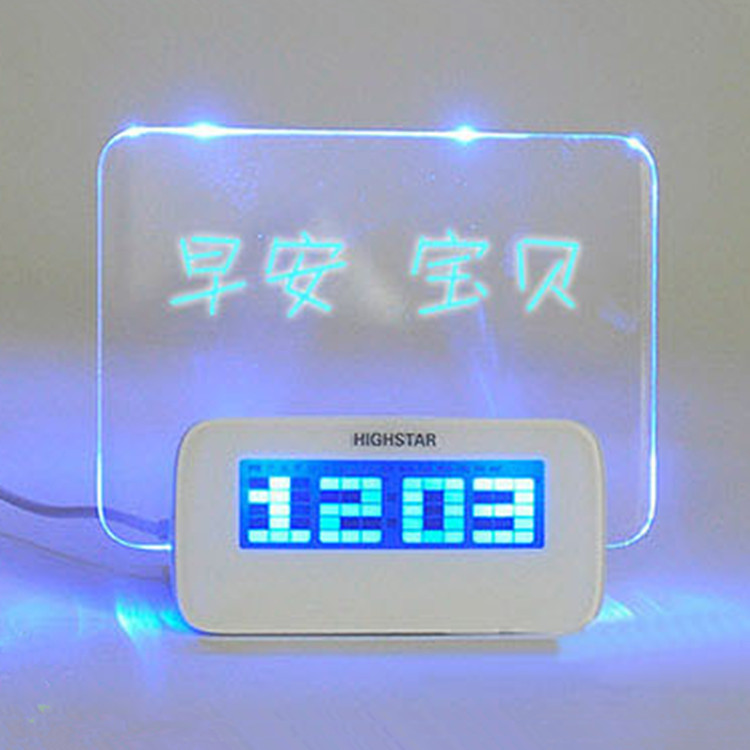In the image, the ground and background are illuminated with a soft blue LED light, giving off a serene atmosphere. Centrally positioned is a large, glass plate with a cable extending from its top. The glass plate is adorned with small LEDs along its upper edge, and features an intricate Asian character etched in light blue. Below this, prominently displayed, is a large, classic white Hopkins and Plattex star. At its center, an LED digital clock reads "12:03", with the numbers glowing in a combination of dark and light blue tones, creating a striking visual contrast.